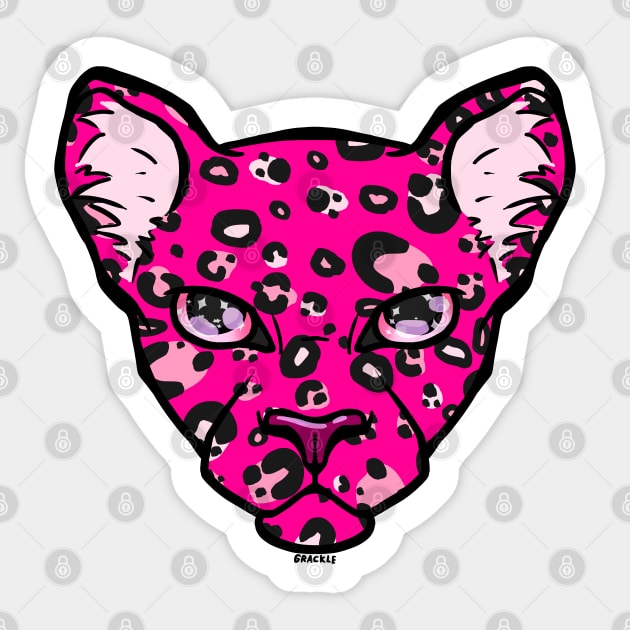In this image, there is a stylized and cartoonish graphic of a bright pink cheetah's face centered against an off-white background with a diagonal grid of gray lock symbols, resembling padlocks or combination locks. The cheetah has a thick white and black border, giving it a sticker-like appearance. The cheetah’s fierce expression features blue stars in its eyes, with a black nose and a bright pink nose tip. Its ears have very light pink tufts of fur, and its fur is adorned with black spots; some spots have white or light pink accents. Below the cheetah’s closed mouth, the artist's name, "Grackle," is prominently displayed. The cheetah, with its intense, starry eyes and stylized design, looks like a mascot or a bold artistic creation.